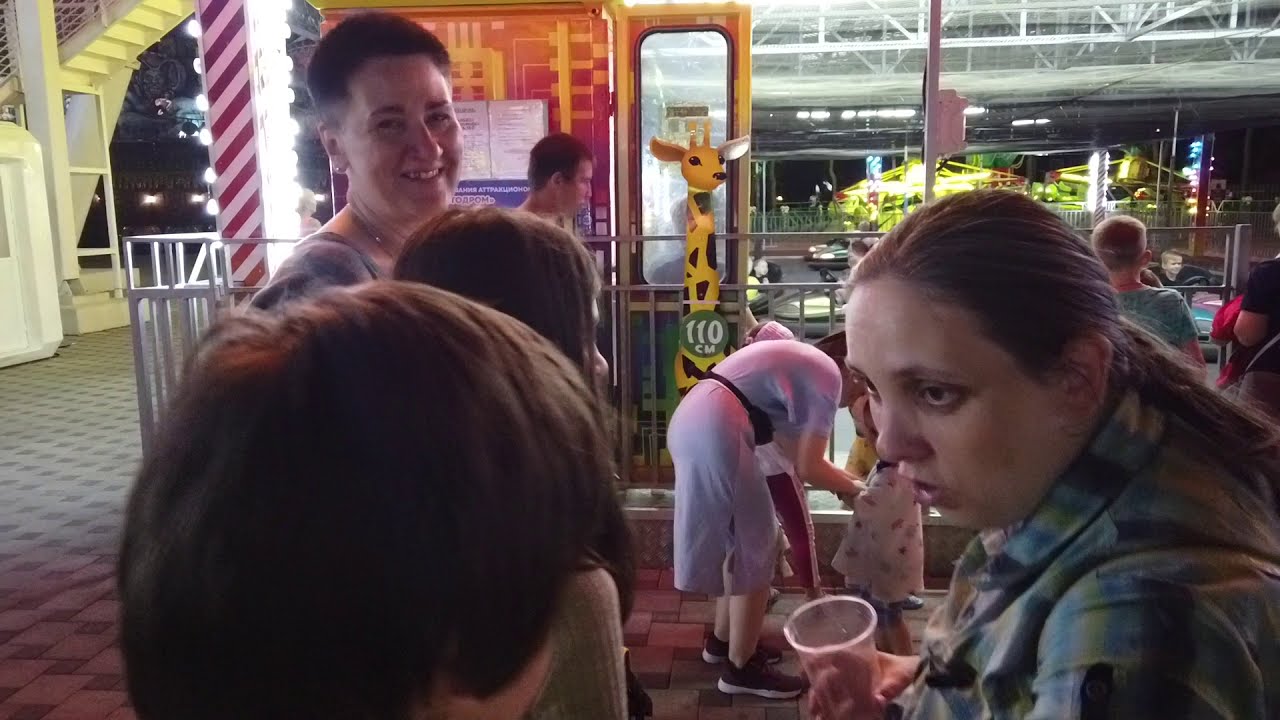This detailed, color photograph in landscape orientation captures a brightly lit shopping mall courtyard, taken at night. The ground is made of stone bricks, setting a textured stage for the scene. Central to the image is a group of people engaging in conversation. Prominently, a woman in the right foreground with her brown hair tied back in a ponytail is pictured in profile, dressed in a blue and yellow checked flannel shirt. She holds a plastic cup, conversing with a boy whose back is turned to the camera.

In the background behind them, a smiling woman with short, dark hair looks directly at the camera. On the top left, another adult catches the viewer's eye while several children are scattered throughout the scene. Adding vibrancy, there is a distinct giraffe toy in yellow and brown with a green tag around its neck, marked "110 centimeters" indicating a height requirement, suggesting the vicinity has games or rides, possibly a fair or amusement park setting.

The image also showcases architectural elements such as a white pedestrian overpass and a staircase in the background, with sunlight filtering into the courtyard beneath the overpass, enhancing the scene's depth with shades of white, gray, brown, tan, yellow, green, silver, and black. The photograph exemplifies representational realism, depicting a lively, bustling environment rich in detail and interaction.